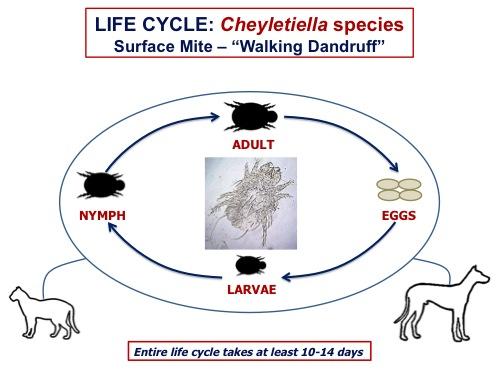The diagram illustrates the life cycle of the surface mite, Chaletiella species, commonly known as "walking dandruff." The title "Life Cycle: Chaletiella species" is prominently displayed at the top in dark blue or black text, with "surface mite - 'walking dandruff'" written below it. The diagram itself is an oval wider than it is tall, depicting the four stages of the mite's life cycle: adult, eggs, larvae, and nymph, each connected by arrows forming a cycle. At the top is the adult mite, followed by the eggs, which are depicted as four small ovals. The eggs lead to the larvae, illustrated by a small bug, which then transitions to the nymph, a slightly larger silhouette, and finally back to the adult mite. At the center of this cycle is a microscope image of the mite, providing a detailed visual reference. Surrounding the oval are silhouettes of a cat and a dog, presented as plain black outlines. A red box at the bottom of the diagram notes that the entire life cycle takes at least 10 to 14 days. The background of the diagram is white, making the details clear and easy to read.